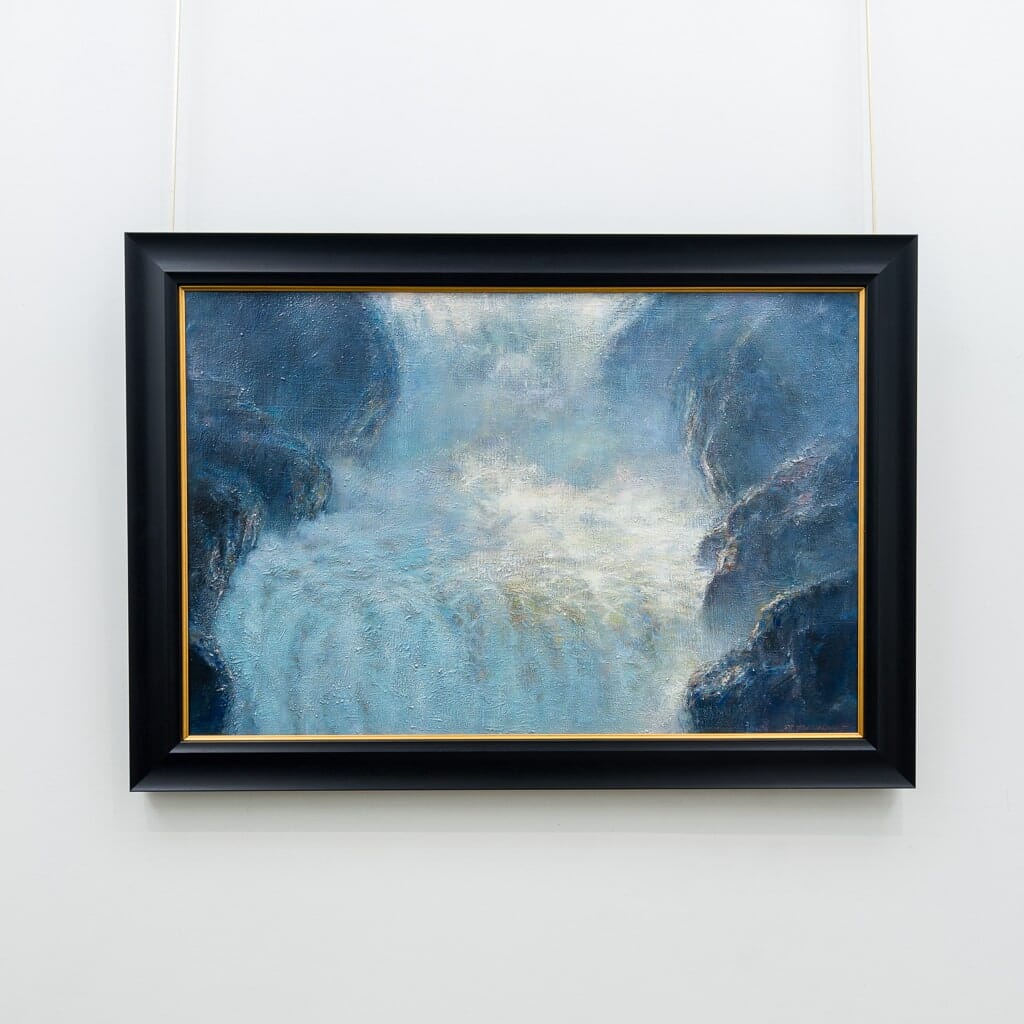The image depicts a horizontal-oriented rectangular painting hanging on a white wall in an art gallery. The painting is encased in a simple black frame with a thin golden inner border, adding a touch of elegance. The frame is suspended by two white strings attached to its top corners. The artwork within the frame is predominantly blue and white, likely an oil painting, portraying a dramatic and abstract depiction of a waterfall. The water appears turbulent and foamy, cascading over a plateau and down onto a lower level, suggesting a multi-tiered waterfall. Flanking this central cascade are rocky cliffs, rendered in darker blues with touches of brown. The painting captures the essence of a mighty waterfall, with the water's movement creating a dynamic and almost mesmerizing visual effect.